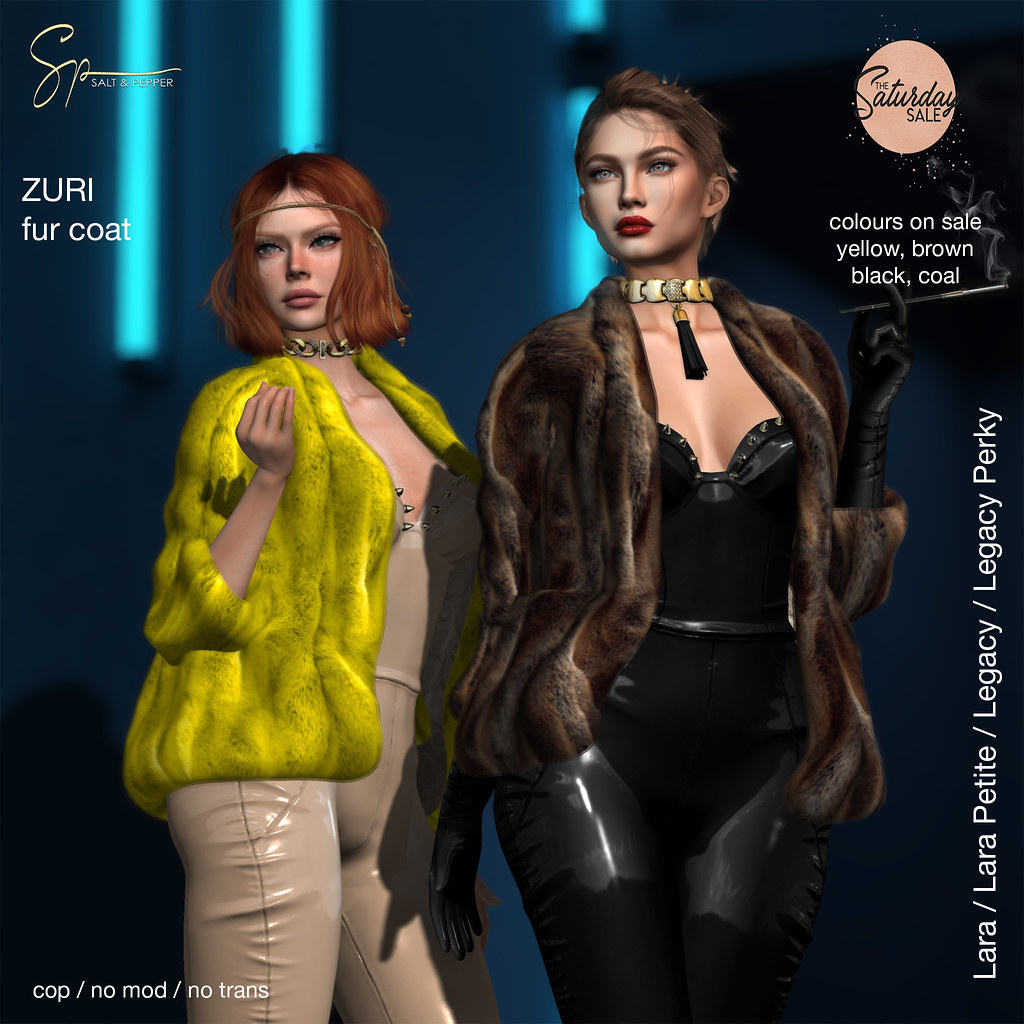This is an advertisement for the video game Second Life, promoting outfits from the Salt and Pepper Zuri Fur Coat collection available in the Saturday Sale. The image features two feminine 3D models against a blue background. The model on the left is dressed in a tan one-piece leather jumper paired with a striking yellow fur coat. The right model sports a sleek black leather outfit complemented by a dark fur coat and swept-back hair. Text details include "Salt and Pepper, Zuri for a coat, cop/no mod/no trans" at the top left, "The Saturday Sale, colors on sale: yellow, brown, black, coal" at the top right, and "Lara/Lara Petite/Legacy/Legacy Perky" running vertically from the bottom left corner. The 3D models, resembling animated mannequins, effectively highlight the advertised outfits' stylish appeal.